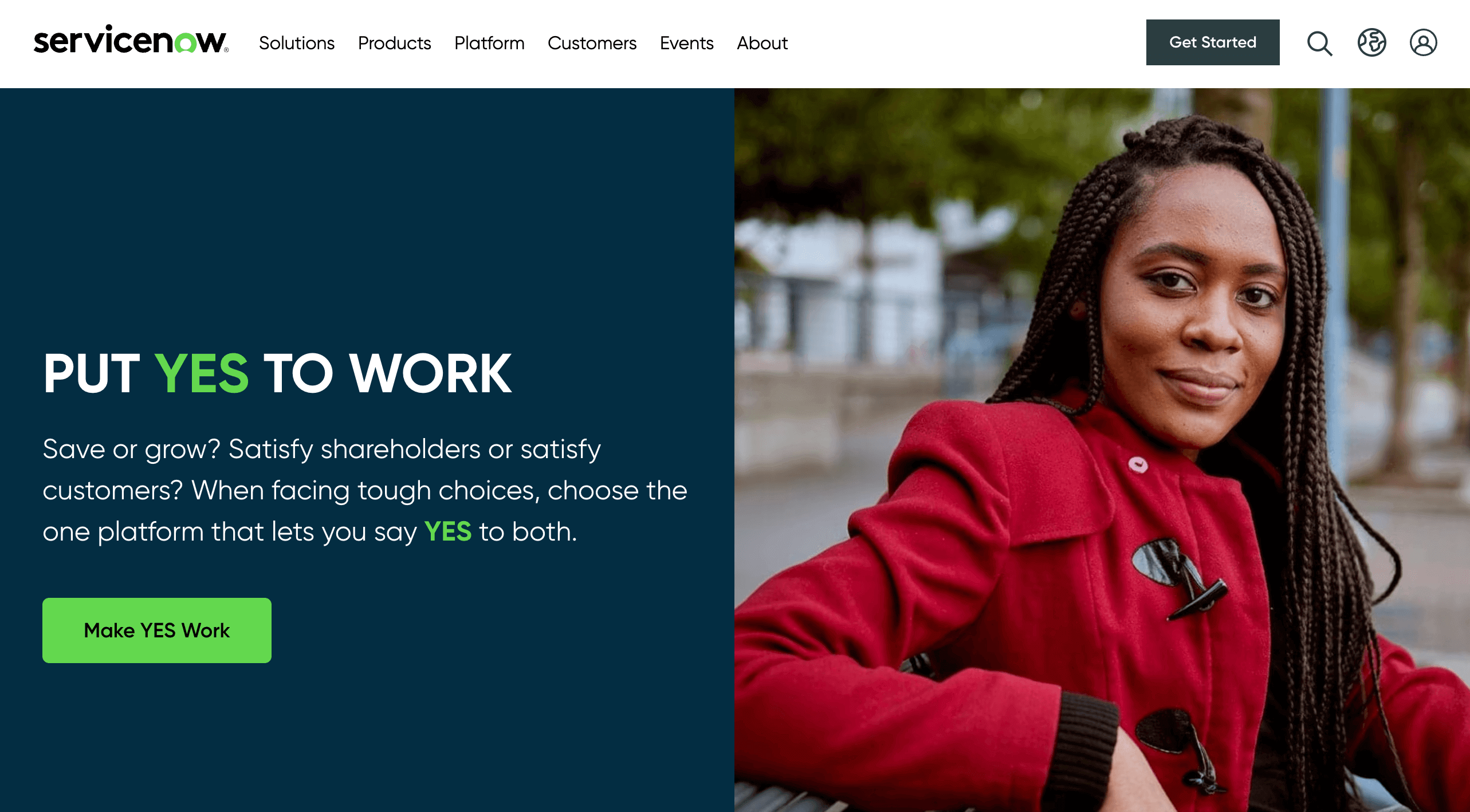Screenshot of a ServiceNow webpage featuring a predominantly white background. At the very top, there's a black and green logo on the left side, displaying "ServiceNow." Adjacent to the logo is a horizontal menu bar with black font that includes the following options: Solutions, Products, Platform, Customers, Events, and About. On the right side of the menu bar, there's a black "Get Started" button with white text, followed by a search icon and two additional icons, possibly for Profile and another function.

Beneath the menu, there's a spacious white area, followed by the main content of the webpage. On the left side of this main section, there's a blue text box featuring the headline "Put Yes to Work" in contrasting white and green text, with "Yes" in green. Below the headline, there's a short paragraph comprising two to three sentences, including phrases like "Save or Grow, Satisfy Shareholders or Satisfy Customers." At the bottom of the text box, there's a green button labeled "Make Yes Work."

Next to the text box, on the right side, there's an image of a woman wearing a red coat. She has braids, and the background of the image is blurred, suggesting an outdoor setting. The woman is smiling confidently at the camera. The page ends with this image.